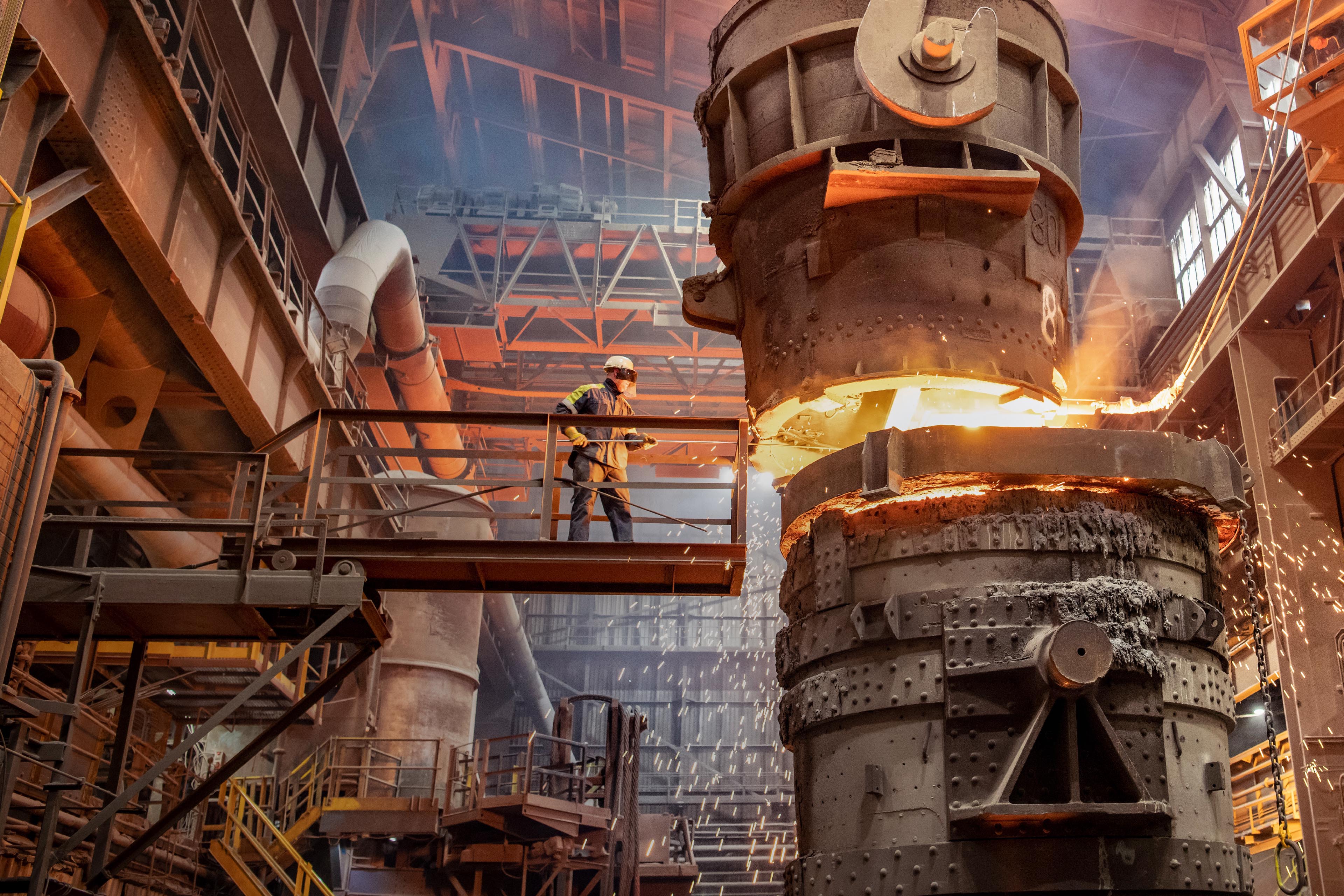The image depicts an industrial scene, seemingly from a video game due to its surreal and intense atmosphere. At its center is a factory interior, with endlessly high ceilings supported by a complex network of gray and brown metal bars. A worker clad in safety gear, including a white hard hat with goggles, yellow gloves, a gray and light green shirt, and blue jeans, stands on a platform that extends from the left side of the image towards the middle. This platform is secured by guardrails, both yellow and brown, and is situated above a series of stairs leading to a lower level.

The worker appears to be manipulating a white stick into bright yellow flames emanating from within a large, vertically aligned mechanical structure. This structure comprises two cylindrical sections, with the lower section showing signs of wear and cracking. The upper section of this machine produces intense light at its center, giving the impression of a powerful industrial process at work. The entire scene exudes an otherworldly and daunting aura, with the grandeur and intimidating complexity of the machinery contributing to its strikingly surreal and dramatic appearance.